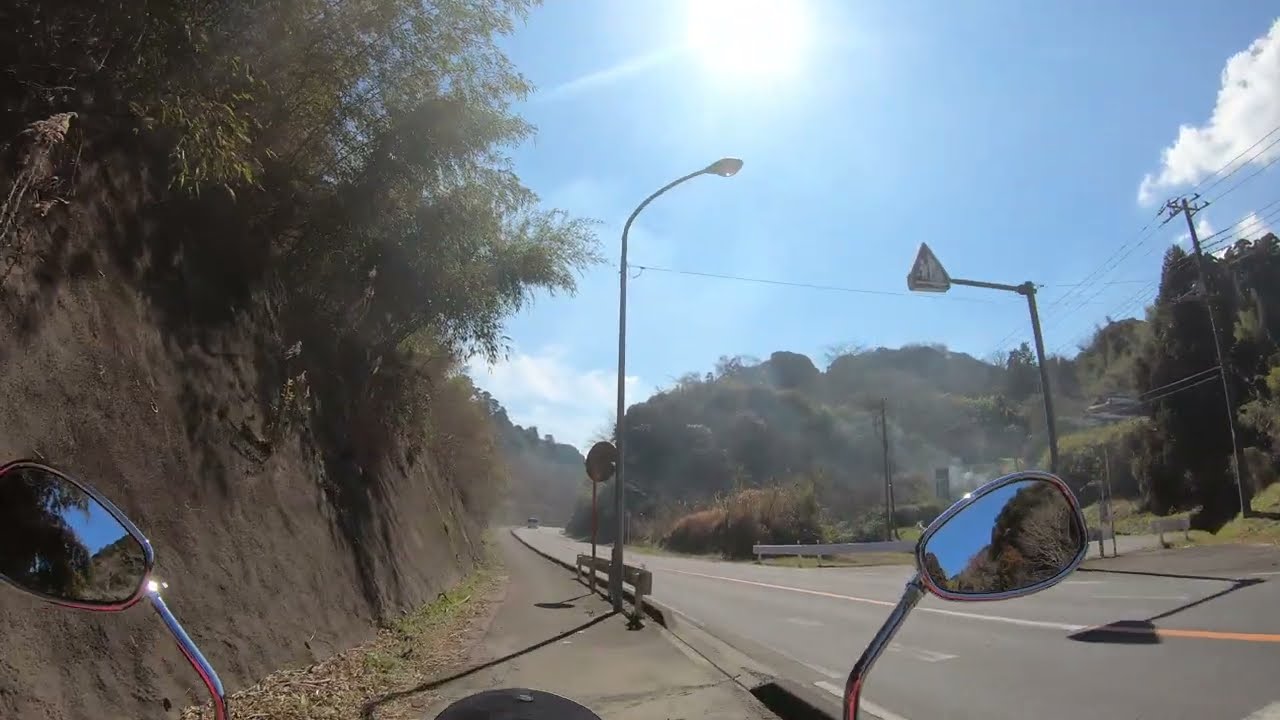In this captivating first-person view photograph, captured from a GoPro-like device mounted on a motorcycle, the viewer is presented with a scenic roadway slicing through a heavily wooded area. The narrow, single-lane, paved road is lined with dense trees, giving the impression that it was meticulously carved out of the surrounding forest. The motorcycle itself is largely out of frame, save for its prominent, high-set rearview mirrors that reflect the verdant foliage behind. The rider appears to have pulled over onto what looks like a sidewalk to the left of the road. The richly blue sky, adorned with a few scattered clouds and a glaring sun at the top center, illuminates the entire scene. On the right side of the image, a streetlight and an electrical cable are visible, along with a distant stop sign peeking through the trees. The photograph details not just the tranquility of this back-road haven but also hints at the sporadic presence of human infrastructure, making it a serene yet subtly dynamic capture.